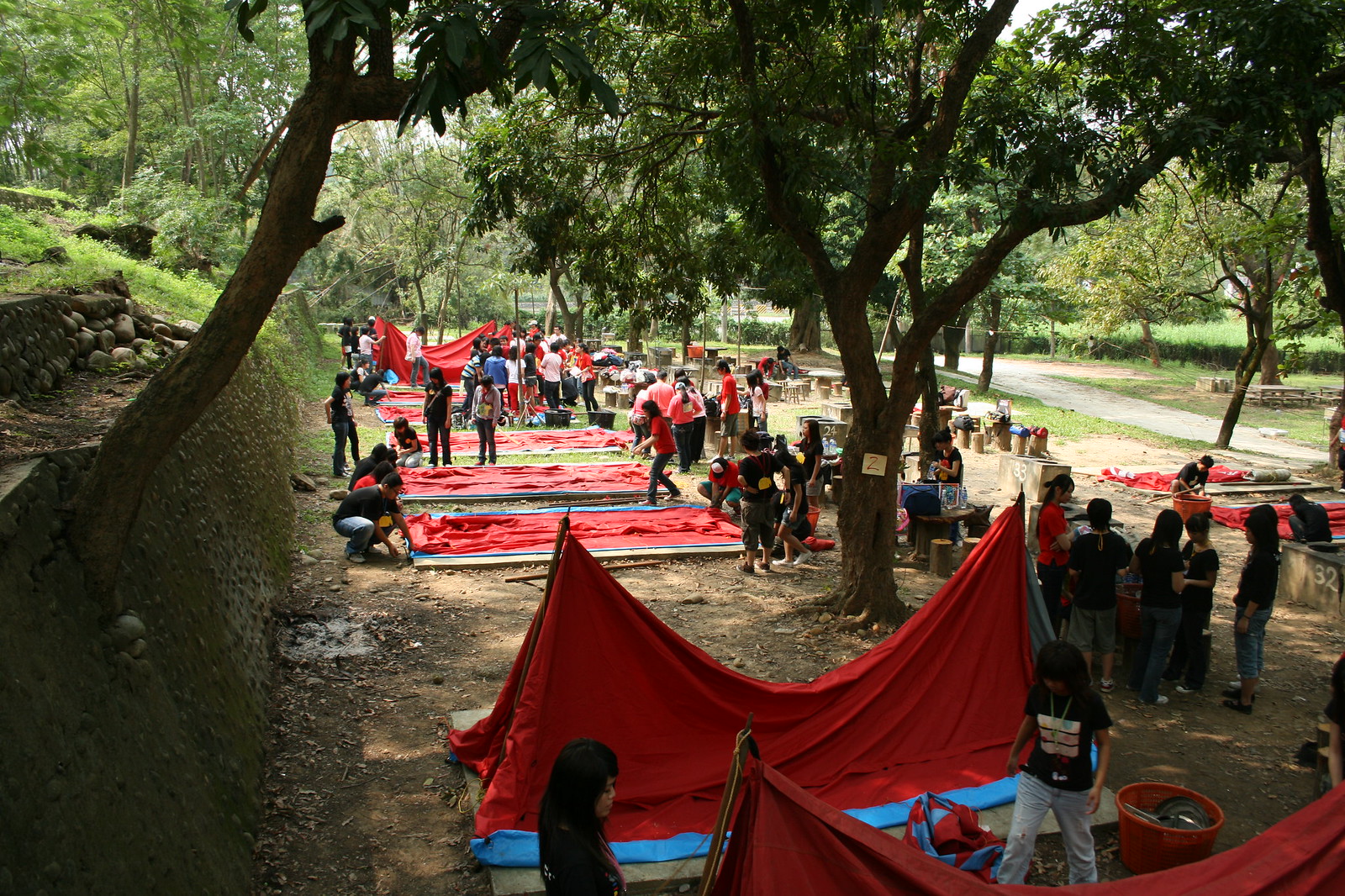In a scenic woodland park, groups of children and adults, predominantly wearing black t-shirts and denim pants, are busily setting up camp. The scene centers around a dirt path flanked by leafy green trees with brown bark. Bright red tents with blue trim at the bottom are scattered across the ground, some fully pitched while others lie flat. Participants work together to raise the tents, signifying a coordinated gathering, possibly a youth group event. The setting is marked by a rock wall from which additional trees and greenery sprout, creating a layered natural backdrop. A sign on a pathway tree, though illegible, further denotes the organized nature of the event. The primary colors in the scene—black, green, red, and blue—add to the vibrant, communal atmosphere at the campsite.